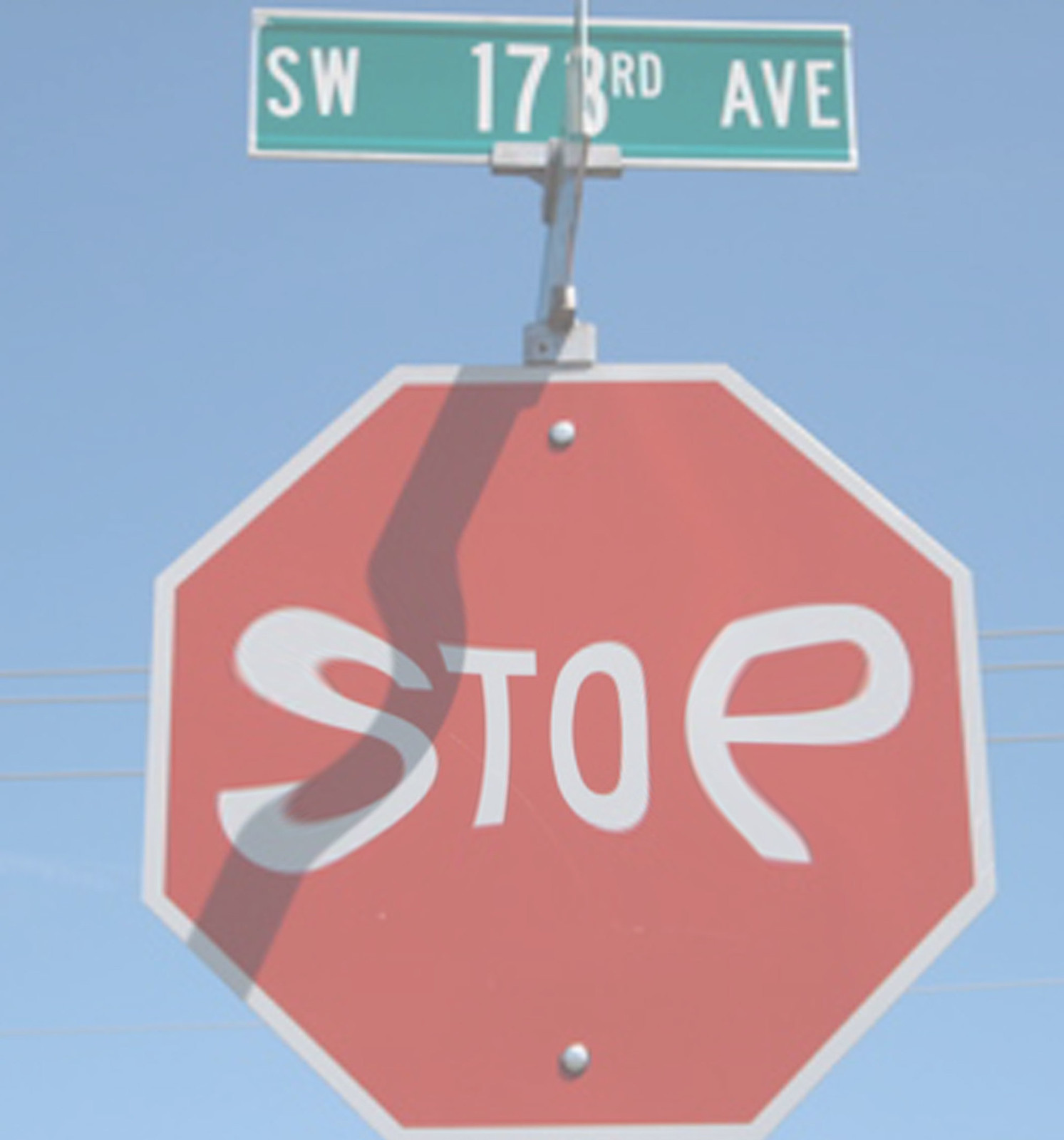This is an edited photograph of a stop sign against a clear, plain blue sky, creating a warped, somewhat hazy effect. The octagon-shaped stop sign, with its red background and white outline, prominently features the distorted and drippy white letters spelling "STOP," with the outer letters "S" and "P" appearing more twisted and enlarged compared to the inner "T" and "O." Atop the stop sign is a green, rectangular street sign reading "Southwest 173rd Avenue," which is bordered by a silver lining. This street sign casts a shadow on the stop sign below, although the warped nature of the stop sign distorts this shadow. In the background, horizontal power lines stretch across the image, adding an additional layer of detail to the outdoor daytime scene.